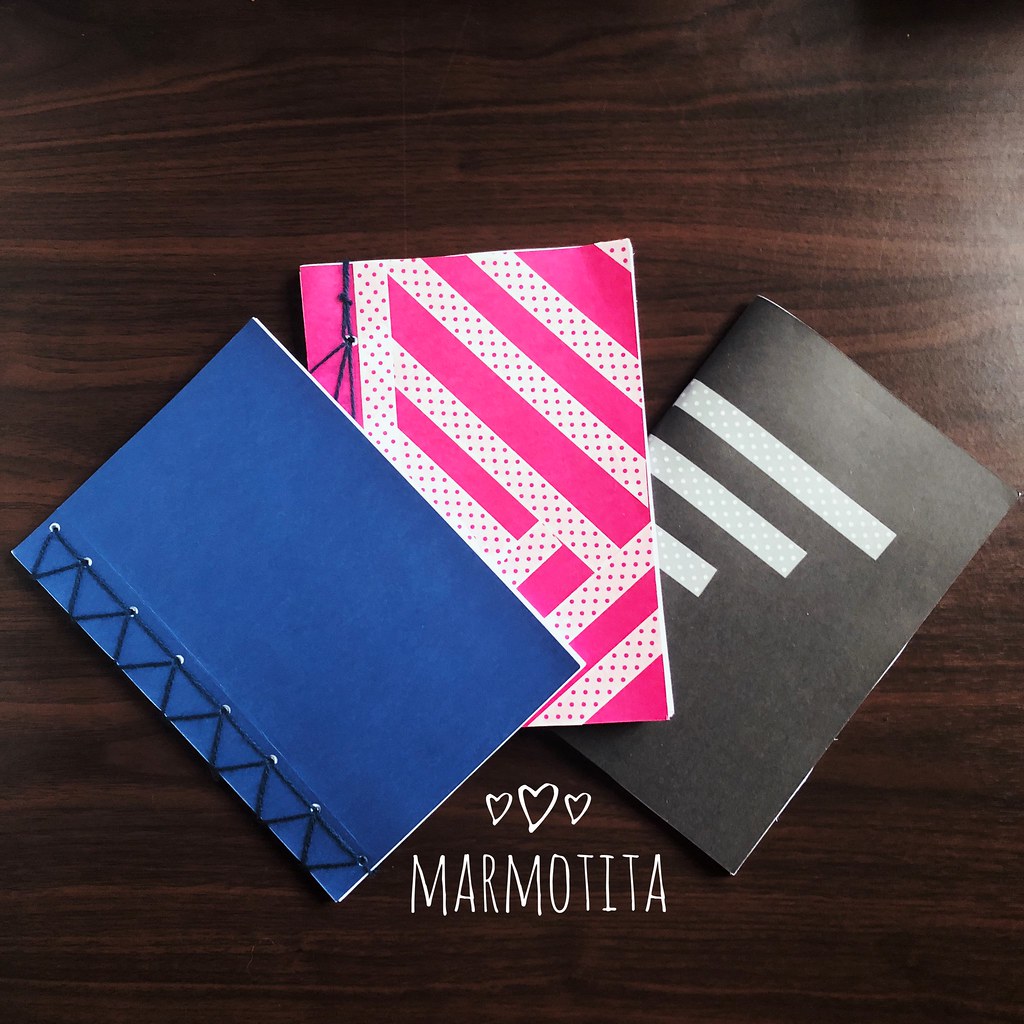The image shows three notebooks placed on a dark wooden table. The notebook on the left has a blue cover with silver rivets and is bound with a black string. The middle notebook features a pink cover with white polka dots and stripes, also tied together with string and featuring a silver rivet. The notebook on the right has a black cover with horizontal gray stripes adorned with white polka dots and appears to be staple-bound. Below the middle notebook, there is a watermark consisting of three handwritten hearts and the word "Marmotita," written in a thin white outline that resembles pencil or pen. Light from the table reflects on the right side of the image.